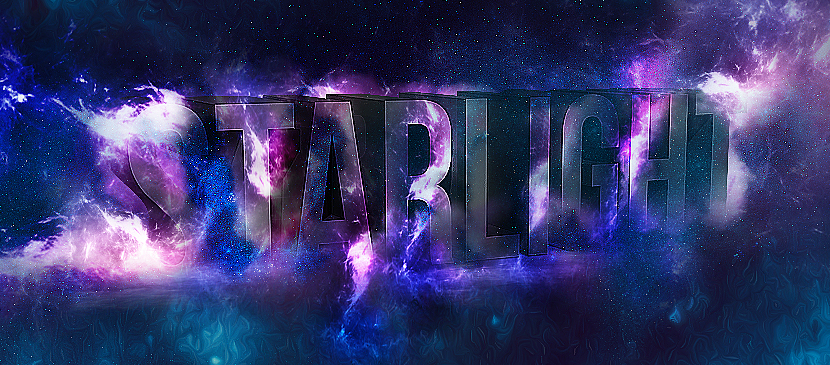The image showcases the word "STARLIGHT" prominently in the center, rendered in all capital letters with a heavy drop shadow giving it a three-dimensional appearance. The text is engulfed in vibrant flames and smoke, emphasizing the letters "S" and "T" which are almost completely covered in intense magenta flames. The background is a dynamic blend of a night sky and psychedelic elements, featuring star-like white specks, gas clouds, and a plethora of colors including blue, purple, pink, turquoise, and magenta. The scene evokes a sense of cosmic chaos, as if "STARLIGHT" has been dropped into a turbulent ocean or a fiery nebula, creating a violent, explosive splash. The entire image is wider than it is tall, with a slightly diagonal orientation of the text, conveying a dramatic, otherworldly atmosphere suitable for a graphic design enthusiast intrigued by space and cosmic phenomena.